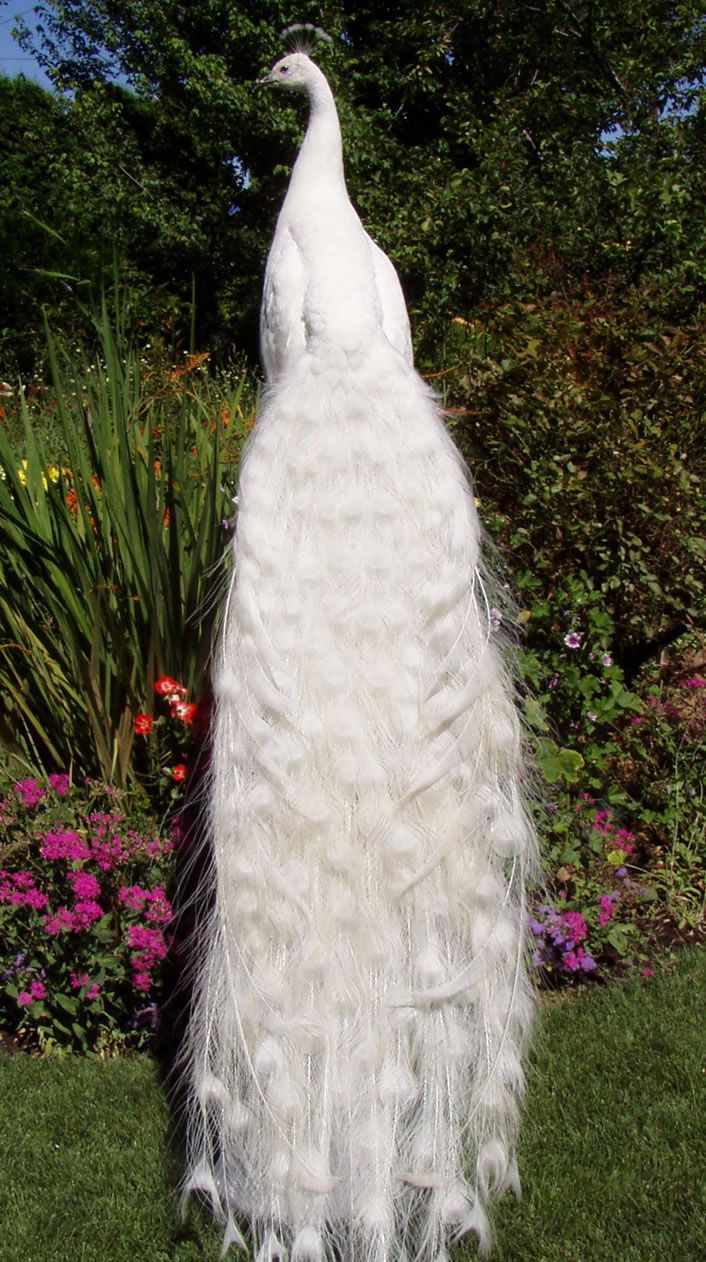In this realistic, vertically oriented photograph, a majestic white bird with an extraordinarily long tail dominates the scene, standing centrally in what appears to be a vibrant garden. The bird, reminiscent of an entirely white peacock or a swan with an extremely extended tail, boasts a tail that stretches nearly three to four times the length of its body, cascading downward in lush, detailed feathers. The bird faces left, giving us a clear view of its elegant tail. 

Surrounding the bird is a lush garden, rich with varied flora. Tall bushes and trees frame the grassy area where the bird stands. The garden is adorned with an array of colorful flowers including red, yellow, purple, and dark pink blooms, adding splashes of color to the predominantly green setting. The sky in the backdrop hints at a sunny day, casting a natural light over the entire scene. The bird’s head is detailed with small black and grey feathers, adding to its intricate appearance. Overall, the photograph captures the serene beauty and grace of the bird amidst its beautiful, natural surroundings.